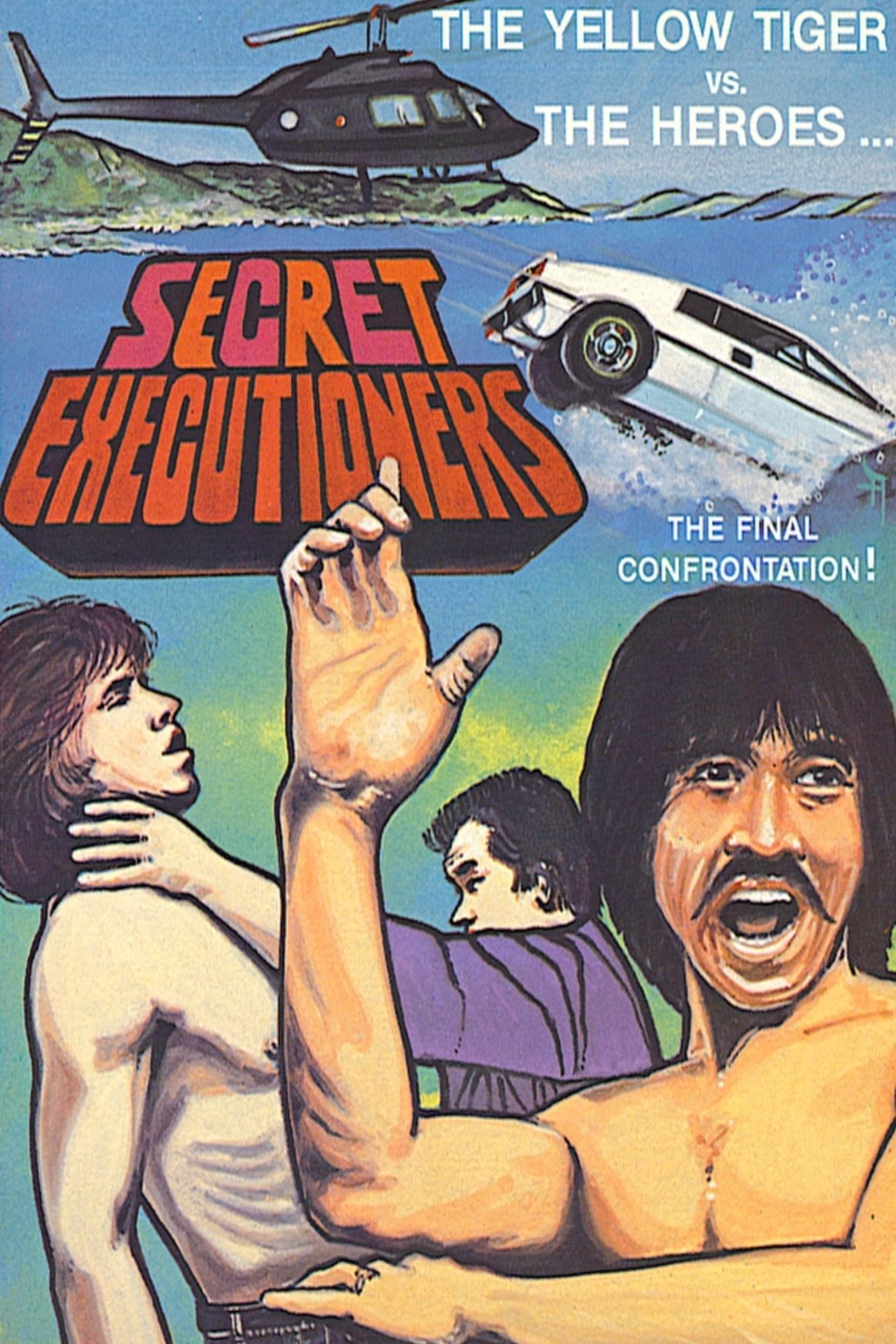This image appears to be a stylized, digitally or traditionally created artwork reminiscent of an old-school Kung Fu movie poster or comic book cover. Dominated by hues of blue, the scene presents a vibrant and dynamic composition. At the top, a brown helicopter flies over a body of water with green hills in the background. Adjacent to the helicopter is the text "The Yellow Tiger vs. The Heroes" in a bold, distinctive style. Just below the helicopter, to the right-hand side, a white car plunges headfirst into the ocean.

Text in large, bold red lettering, "Secret Executioners," is positioned to the left of the car, while beneath the car, in white text, is "The Final Confrontation." The lower part of the image features an intense scene with caricatures of three men. On the left, an individual is being choked by another man dressed in purple with one hand around his throat. In the foreground, an Asian man with long black hair, a mustache, and a Kung Fu stance yells with his mouth wide open. The overall style, with its vibrant color palette and dynamic action, gives the image an older, vintage comic book or film poster feel.